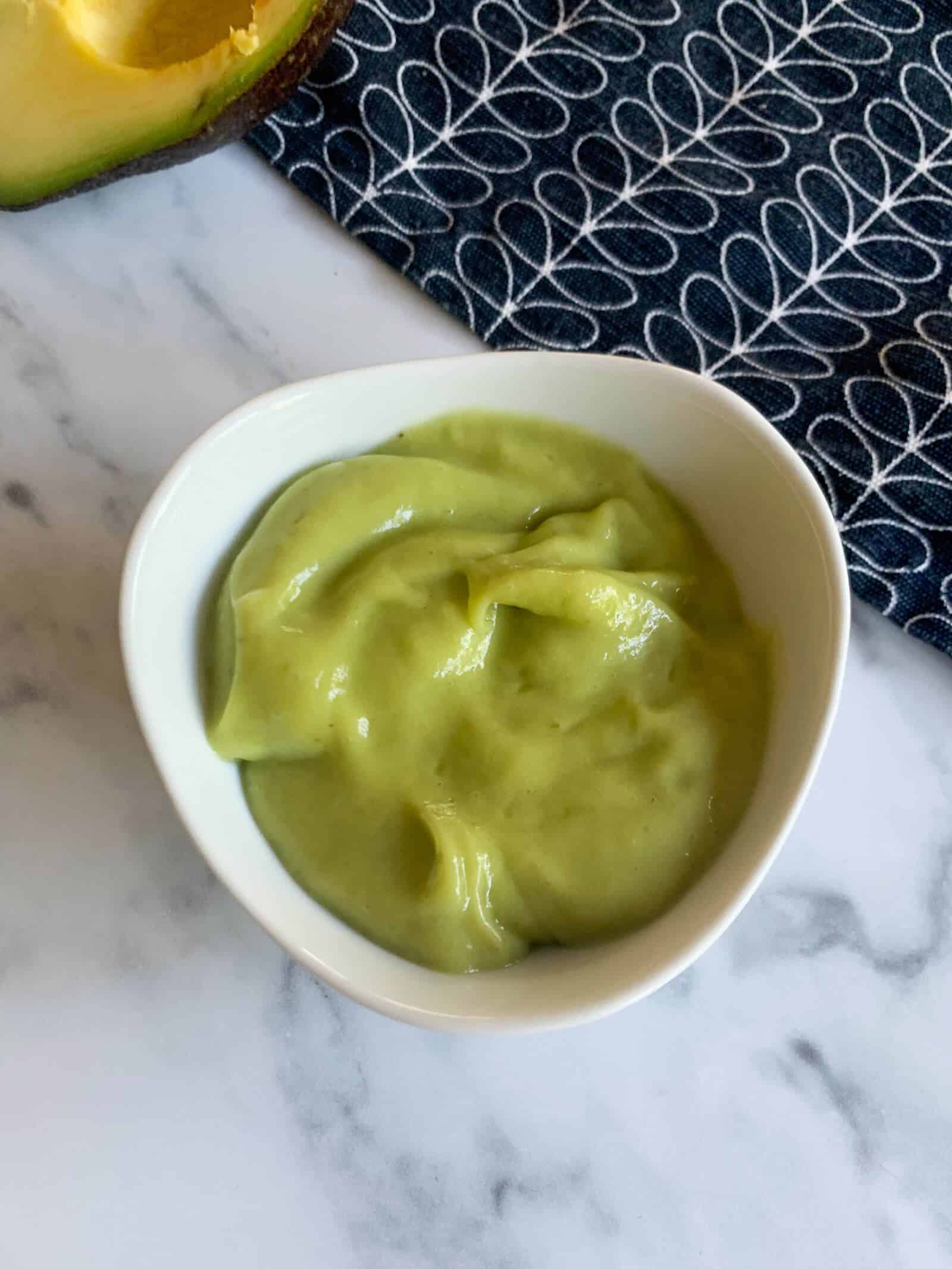This image showcases a homemade guacamole dip with a very smooth, almost liquid consistency, presented in a uniquely shaped white bowl with three rounded edges. The bowl is centrally placed on a white and gray marble countertop, which features intricate veining in darker blacks and grays. In the top left corner of the image, there is a half avocado with the pit removed, suggesting it was used to prepare the guacamole. Additionally, a black kitchen towel adorned with white looping patterns, which resemble butterflies, lies on the countertop in the upper right part of the photograph, extending over part of the marble surface. The overall scene combines elements of culinary preparation with a striking kitchen aesthetic.